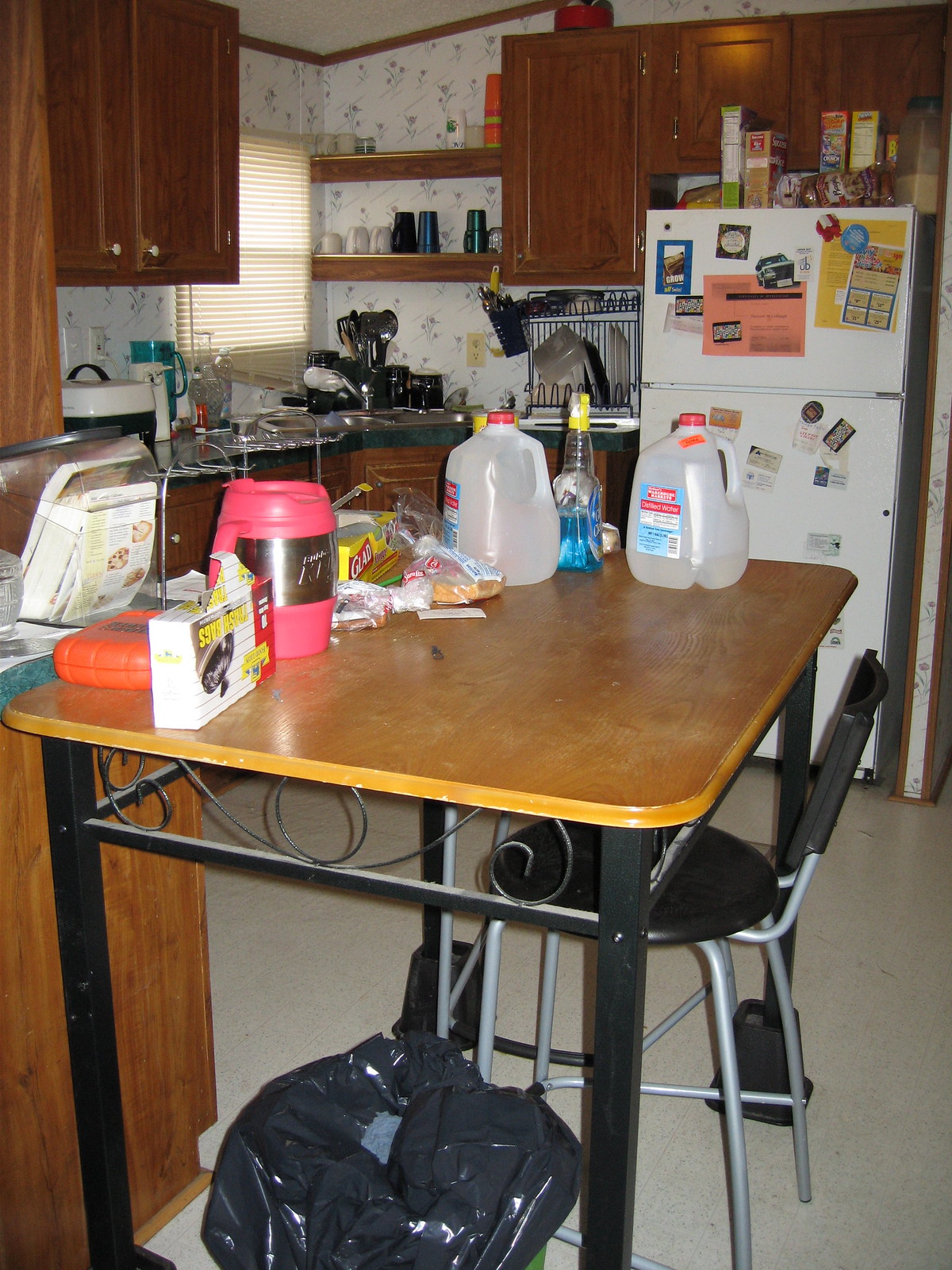In the image, a cozy kitchen setting is depicted. At the center is a small dining table with a walnut brown wood tabletop paired with black steel chairs, one of which has gray-colored legs and is tucked neatly underneath the table. Atop the table sit two empty jugs, a spray bottle containing blue liquid—presumably window or glass cleaner—and a small pink tub with indistinguishable writing.

The kitchen boasts a white refrigerator and a black stove with a stainless steel top. A wash sink is visible, surrounded by numerous utensils including spoons. Above the sink, dark brown cabinets line the wall, with an estimated count of four. On the left-hand side of the sink is a hot plate with a white cover and a black handle. The open cabinets reveal an assortment of glasses, including green and black ones, alongside various small, unidentifiable items, adding to the homey and lived-in atmosphere of the space.